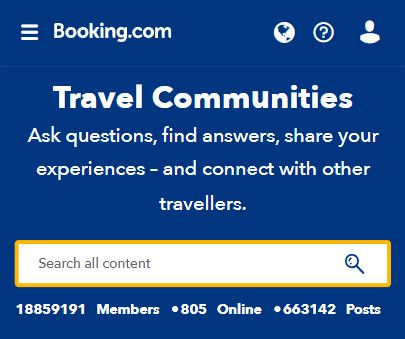**Original Caption Given Using Voice:**
Then it tells us to create a company, so it's bookdn.com, search, it's called QuestionMarketSite, and then there's travel communities, ask questions, find answers, share experiences, and connect with the travelers, book background, and there's info field, search all content, modify glass. Number is 1-885-9191, number is circle 805, online, dot 663142, post, yeah, not very visible, grainy, not much visible.

**Cleaned Up and Detailed Caption:**
The image shows the interface of a new travel-oriented website called "QuestionMarketSite," accessible via bookdn.com. This platform features various travel communities where users can ask questions, find answers, share experiences, and connect with fellow travelers. The background of the webpage showcases a book-themed design, with an informative field prompt and a search bar allowing users to explore all content. Additionally, a magnifying glass icon facilitates the search function. Key contact numbers listed include 1-885-9191 and a secondary number within a circular design, labeled as 805. The online identifier "dot 663142" is also displayed. However, the image quality is quite grainy and not very clear, making some details hard to discern.